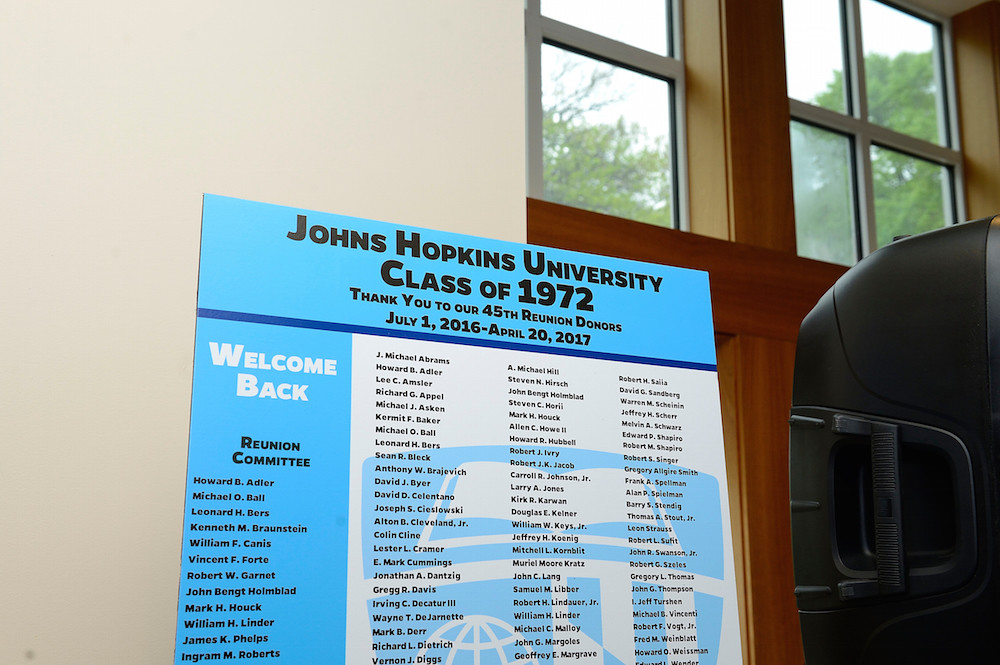This photo captures a large, prominently displayed sign for the Johns Hopkins University Class of 1972 reunion, situated against a wall inside the reunion venue. The sign is predominantly blue and white. On the left portion of the sign, "Welcome Back" is prominently featured, followed by a list of the reunion committee members. This section is presented in blue text. The right side includes an expression of gratitude towards the 45th reunion donors, dated from July 1st, 2016 to April 20th, 2017. The main center section of the sign, which is white, meticulously lists all class members in three columns of black text. At the center of the sign, a blue shield design of Johns Hopkins University is displayed. Surrounded by the sign, the venue features a door and windows on the right side, along with what appears to be a black speaker. The detailed and organized layout of the sign captures the essence of the reunion event and the significant contributions of its attendees.